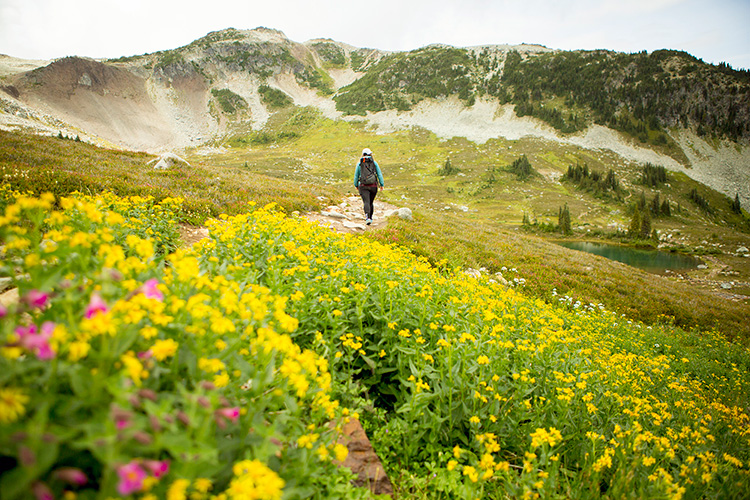This color photograph captures a picturesque landscape with a hiker as its focal point. Set against a backdrop where a light blue sky meets hills covered with green brush, the image showcases the sandy, light brown, and white hues of the hillsides. In the distance, you can glimpse a body of water, possibly a pond or lake, partially obscured by a hill in the mid-ground. Pine trees dot the landscape, adding depth and layers to the scenery.

In the foreground, a rugged, stone-laden dirt path cuts through a vibrant field of flowers, predominantly yellow, with hints of pink on the left side. The path, flanked by green grass, leads away from the viewer, guiding their eyes to the hiker walking away from the camera. The hiker, positioned centrally, is adorned in a blue long-sleeve shirt, dark pants, and a hat, with a visible backpack strapped on their shoulders.

The bottom half of the photograph is enriched by the dense cluster of yellow flowers interspersed with occasional pink blooms on the left, contrasting vividly with the path and greenery. The combined visual elements of rugged terrain, vibrant florals, serene water, and distant hills create a harmonious and captivating scene, encapsulated by the tranquil expanse of the sky above.